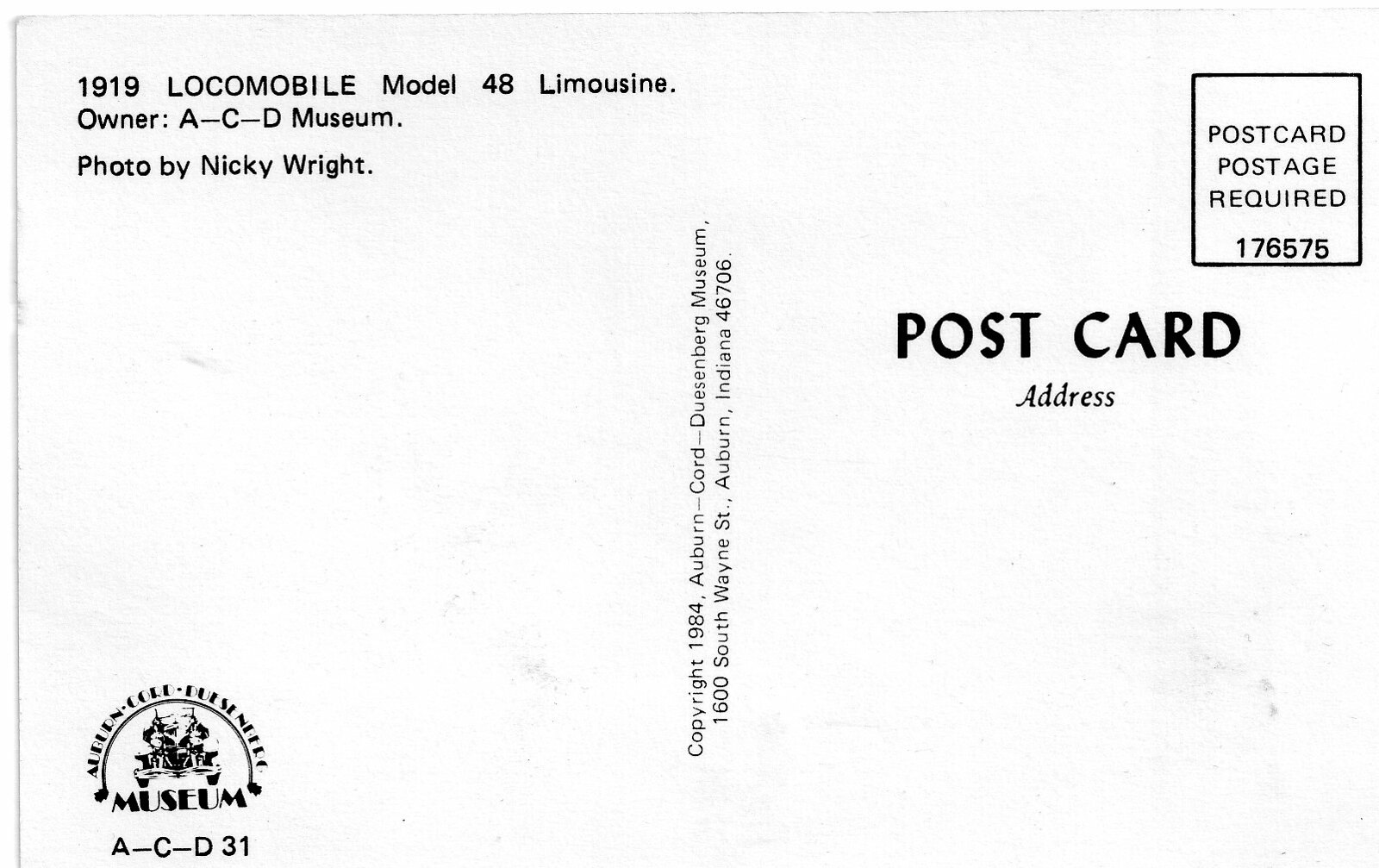The image is a scanned, white postcard predominantly featuring text and a small logo. The upper left corner identifies the postcard with "1919 Locomobile Model 48 Limousine, Owner A.C.D. Museum, Photo by Nikki Wright." Vertically down the center of the postcard, the text "Copyright 1984, Auburn Cord Duesenberg Museum, 1600 South Wayne Street, Auburn, Indiana 46706" is printed. In the bottom left, a logo displays a black and white drawing of a car, associated with the Auburn Cord Duesenberg Museum. The upper right corner includes the instruction for mailing, "Postcard Postage Required 176575" and beneath it, the words "Postcard Address." The postcard shows faint pencil or ink stains, adding a touch of age to the otherwise clean, white appearance.